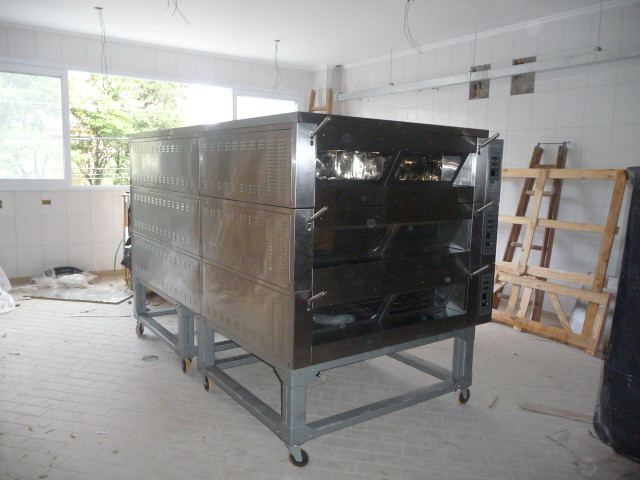The image captures a predominantly white-tiled room, possibly a garage or shop, featuring a large, central rectangular silver object. This object comprises six individual box-like structures, each equipped with clear glass windows and six handles on the user-facing side, allowing a glimpse inside. The silver object rests on a robust steel frame, supported by wheels for mobility. Suspended from the ceiling are several wires, adding to the industrial feel of the space.

Located against the right wall are multiple wooden planks and a stepladder. The room is uniformly white, with large tile squares on the walls and smaller tile pieces on the floor, creating a seamless, bright environment. An open window on the left side bathes the scene in natural light, highlighting the green trees visible outside.